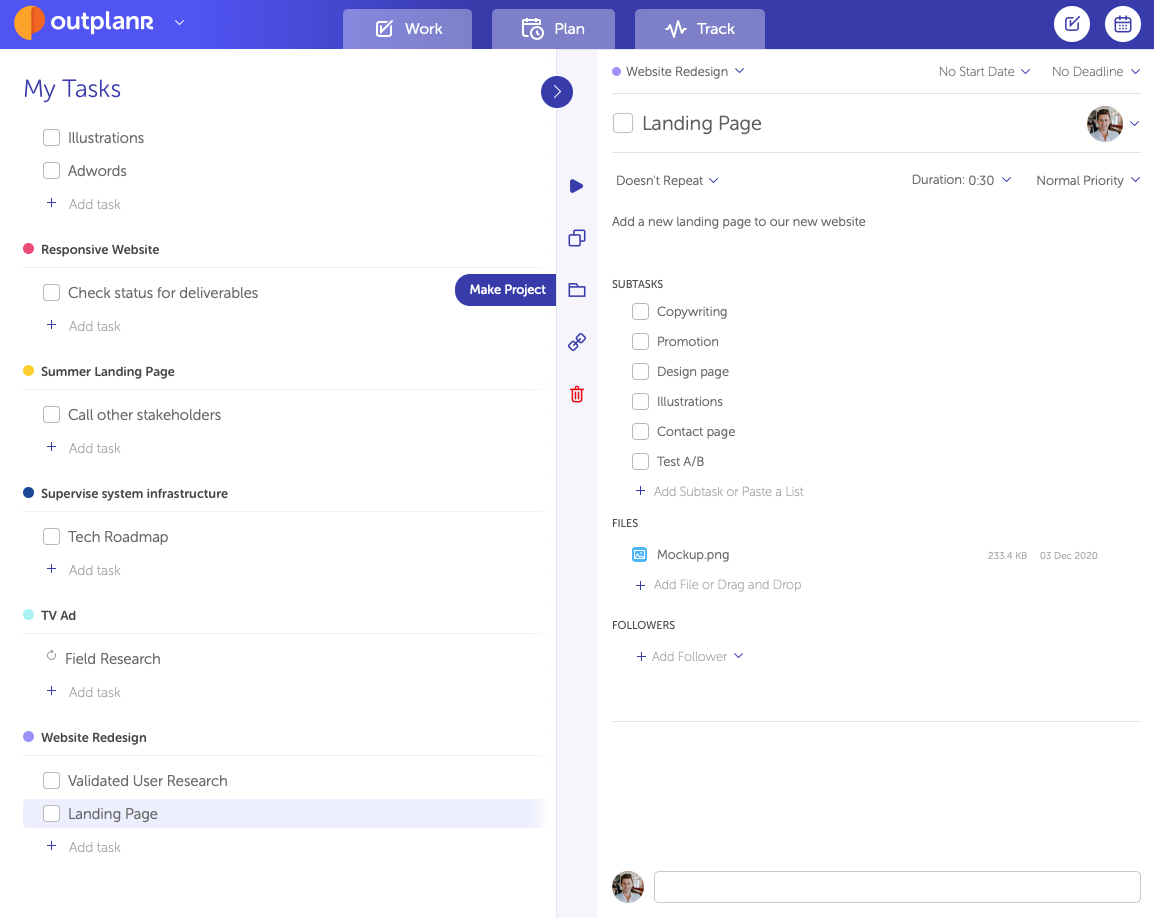The image depicts a detailed view of an individual's work planner desktop interface. At the top of the screen, there's a sleek taskbar with a gradient transition from a light blue-purple on the left to a darker hue on the right. The toolbar features a distinctive logo consisting of a light orange half-circle with a smaller dark orange half-circle attached to it. The logo is accompanied by the brand name "OutPlanR," with the capitalization uniquely placing emphasis on the "R."

The interface includes several tabs labeled "Work," "Plan," and "Track." Adjacent to these, there are two white circle icons—one containing a square with a check mark, symbolizing completed tasks, and another resembling a calendar.

Beneath the toolbar, a section labeled "My Tasks" lists various tasks, none of which have been marked complete. The task list includes:

1. Adworks
2. Responsive Website
3. Check Status for Deliverables
4. Summer Landing Page Call
5. Other Stakeholders
6. Supervised System Infrastructure
7. Tech Roadmap
8. TV Ad
9. Field Research
10. Website Redesign
11. Validate User Research
12. Landing Page

On the right side of the planner, a profile picture of a Caucasian man with short brown hair wearing a white shirt is displayed. Below his image, the task "Landing Page" is highlighted. This task is detailed as not repeating, with a duration set to 30 minutes and marked as normal priority.

The highlighted task includes several sub-tasks:
- Copywriting
- Promotion
- Design Page
- Illustrations
- Contact Page
- Test A/B
- Files
- Mockup PNG

An option for "Followers" is provided, though none are listed. In the center of the page, a red rubbish bin icon is prominently displayed. The taskbar includes more icons such as a play button, a copy button, a folder, a link button, and another rubbish bin.

The overall interface appears systematically organized, aiming to optimize productivity through its well-structured task management features.